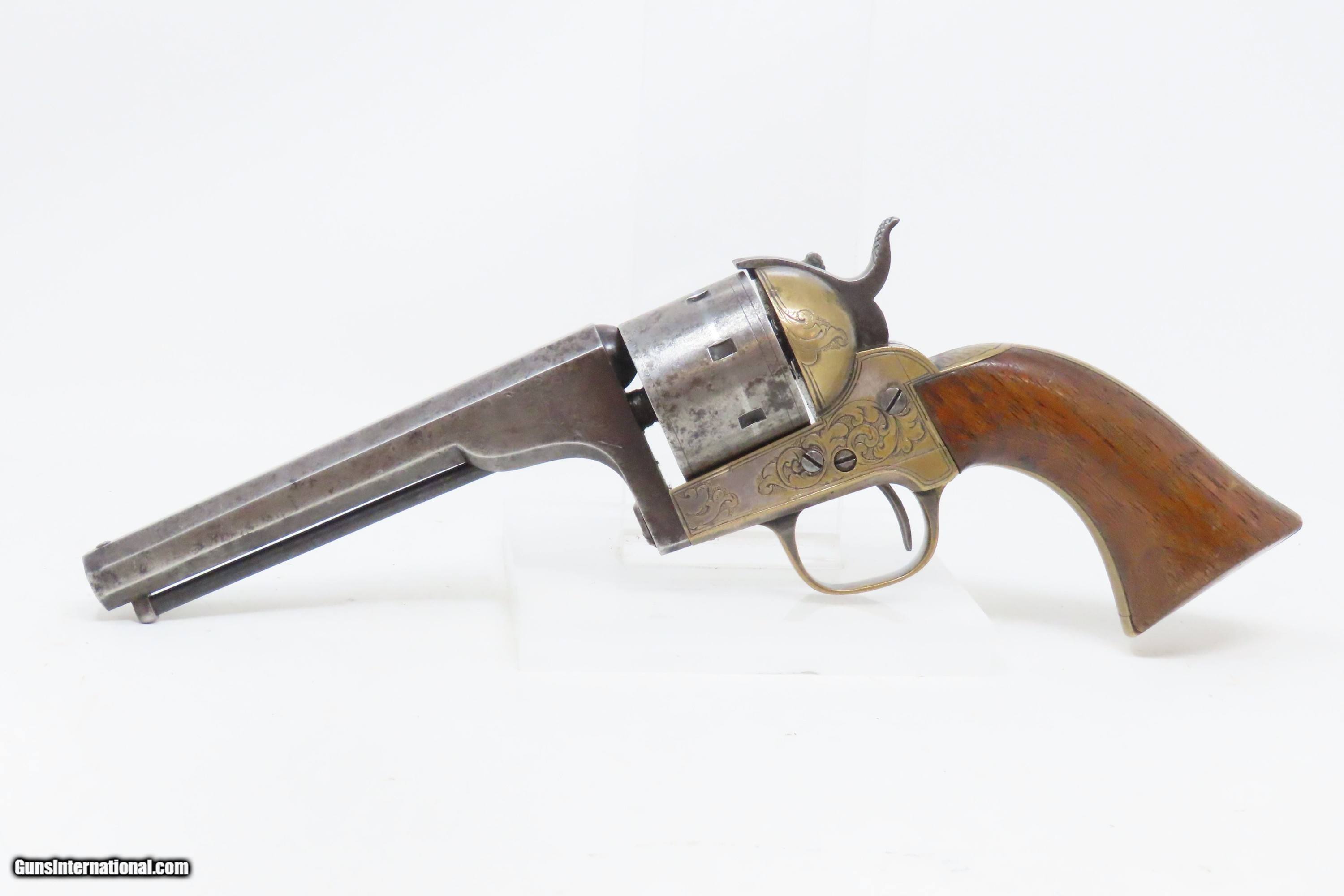The photograph depicts a vintage western revolver with a wooden handle, positioned on a pristine white background. The well-worn pistol, likely an auction item, rests on a clear display base, highlighting its rustic charm and historical significance. The barrel, trigger, and bullet chamber are crafted from metal, with a silver sheen that has succumbed to rust over time, suggesting a long and storied past. Intricate scroll-like designs are etched into the gold-toned metal near the trigger, adding a touch of artistry to its rugged appearance. Silver screws secure the handle to the body of the revolver, further emphasizing its detailed craftsmanship. In the bottom left corner of the image, "gunsinternational.com" is clearly watermarked in white text outlined in black, indicating the source or featured listing of this classic firearm.